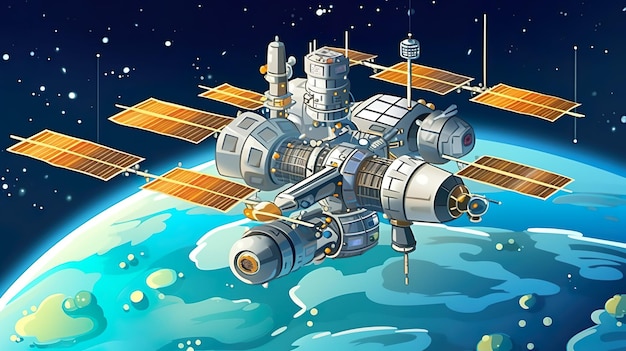The image appears to be a computer-generated or cartoon-style depiction of a large, complex space station in orbit around a planet, likely Earth, which is partially visible at the bottom and right side of the image. The space station itself features a unique zigzag configuration composed of interconnected capsules, adorned with numerous gold-colored solar panels and circular windows. It also has a multitude of needle-like protrusions and dome-shaped structures, giving it an intricate and somewhat industrial appearance. The planet below is illustrated with blues, greens, and random blob-like designs, representing land and water. The background is a dark, star-studded expanse with white dots symbolizing stars scattered throughout the black sky.